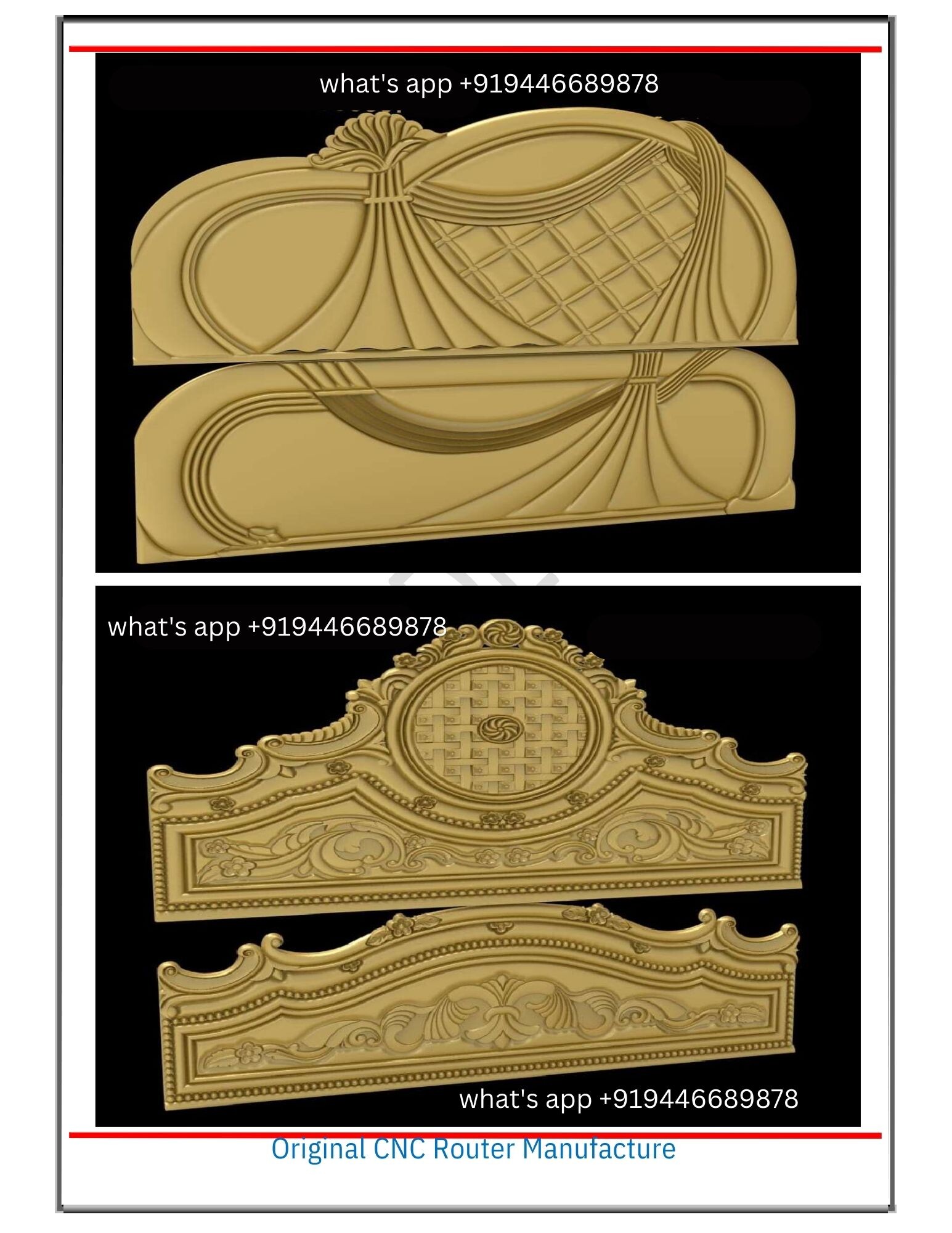This image consists of two color photographs displayed in a portrait orientation, each showcasing ornate gold headboards and footboards against a black background. Both photographs are framed by a white border with a thin black rule.

The top half of the image features a headboard and footboard, crafted with a shiny gold finish. The headboard displays a wavy, draped fabric motif on the right side, complemented by a checkered print underneath, and a cluster of flowers on the left. The footboard mirrors the headboard's opulence with a horizontal top partially draped with fabric on the right, but lacks the central flower cluster. 

The bottom half of the image shows another pair of gold headboards and footboards, designed with a similar artistic flair. The headboard has a prominent ellipse in the center flanked by elaborate scrollwork running along the edges and slanted tops, with additional scrolling below. The footboard continues this sophisticated design but without the central ellipse.

White text in both sections reads "WhatsApp +919446689878," and at the very bottom, in blue text, it states "Original CNC Router Manufacturer." Both headboard images are presented in a photographic representational realism style, highlighting their intricate floral and fabric-like patterns.